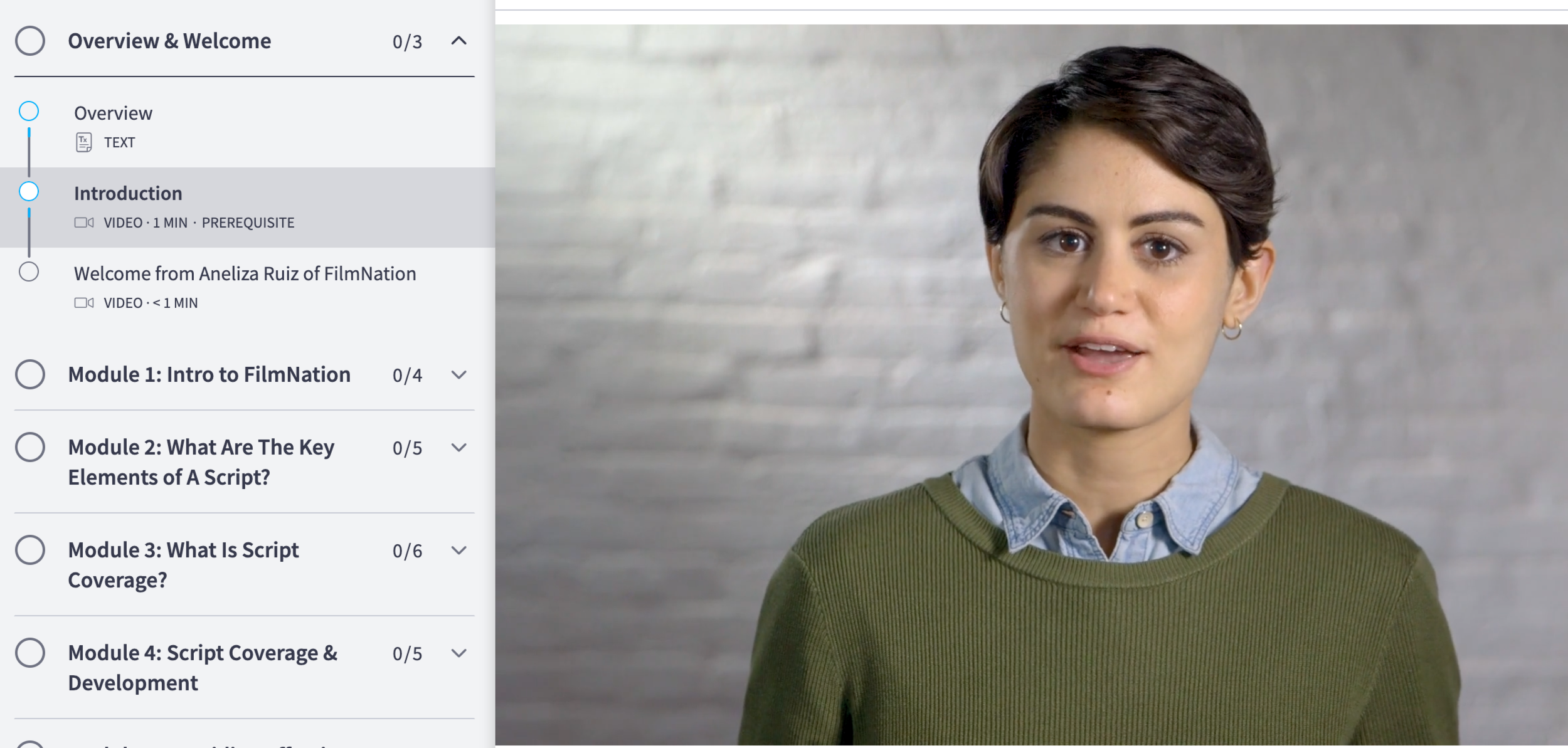A screen capture showcasing an online presentation in a slideshow format. 

On the left third of the screen, there is a vertical arrangement of bulleted points and various highlighted elements. At the top of this column, a radio button is labeled "Overview and Welcome," which is followed by '0/3'. Below this, other radio buttons show additional content sections: "Overview," "Introduction," and "Welcome from Aneliz Arize of Film Nation," with a corresponding three-minute introductory video marked as a prerequisite, appearing highlighted in light gray. The sections continue with "Module 1: Intro to Film Nation" labeled '0/4', "Module 2: What are the Key Elements of a Script?" labeled '0/5', "Module 3: What is Script Coverage?" labeled '0/5', and "Module 4: Script Coverage and Development," also labeled '0/5'.

On the right two-thirds of the screen, there is a video still that appears to be the start of the introductory video mentioned earlier. The video features a young woman, likely in her early 30s, with brunette hair and fair complexion. She is wearing a green sweater over a blue shirt and standing against a white brick wall, looking straight ahead with her mouth slightly open, as if in mid-sentence.